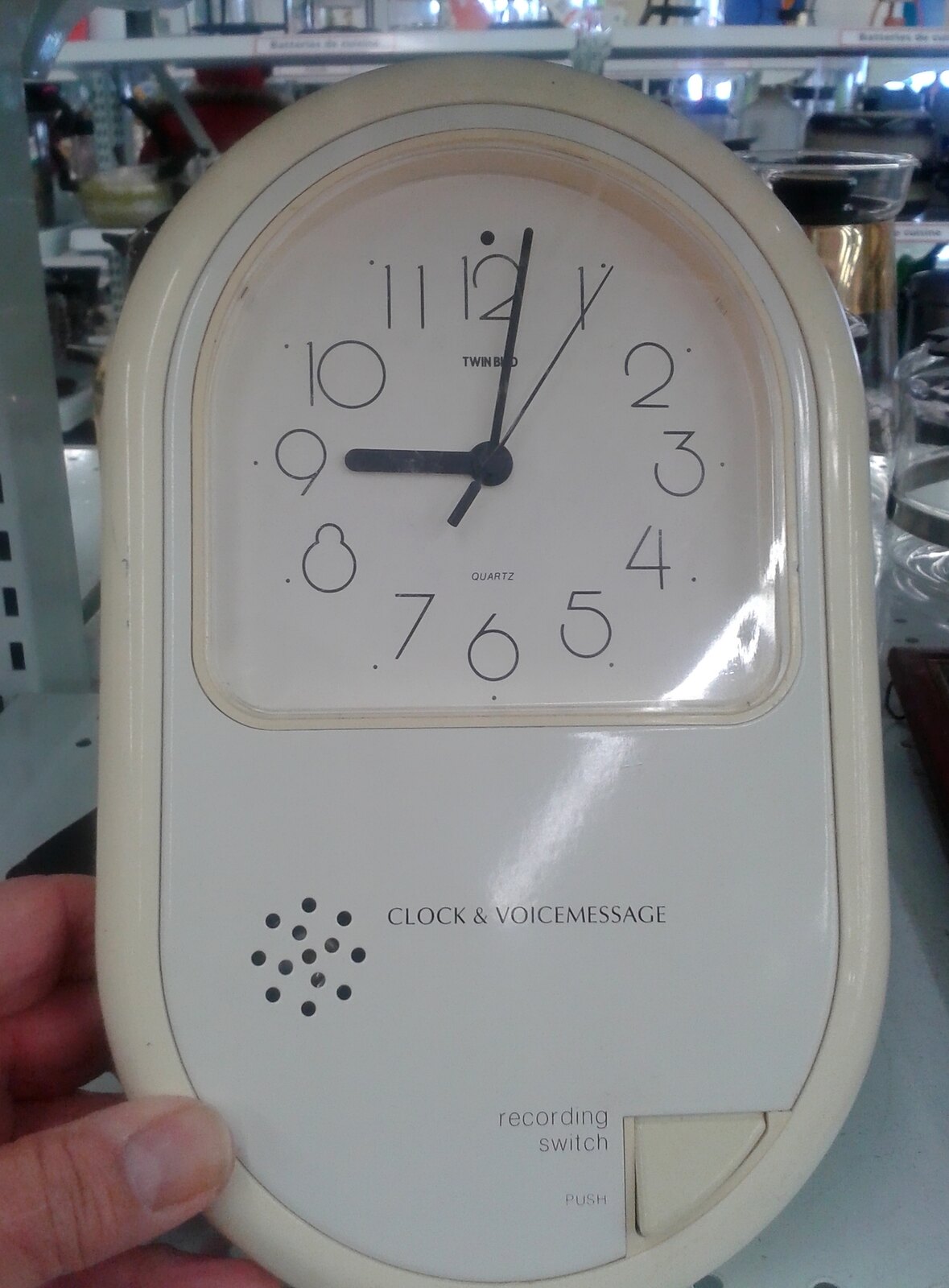A close-up photograph captures a well-worn, oval-shaped clock held delicately between the thumb and fingers of a person with white skin, using their left hand. The clock, made of white plastic, exhibits signs of aging and discoloration in certain areas. The upper half of the device is dedicated to the clock face, which is white with bold black numerals and matching black hour and minute hands. A slender black second hand also ticks away the time. Below the clock face, the words "Clock" and "Voice Message" are printed, alongside a perforated speaker area. At the bottom end of the device, a cream-colored button labeled "Recording Switch - Push" is visible. The background reveals various items for sale displayed on tables and shelves, suggesting that the scene is set at a bustling flea market.